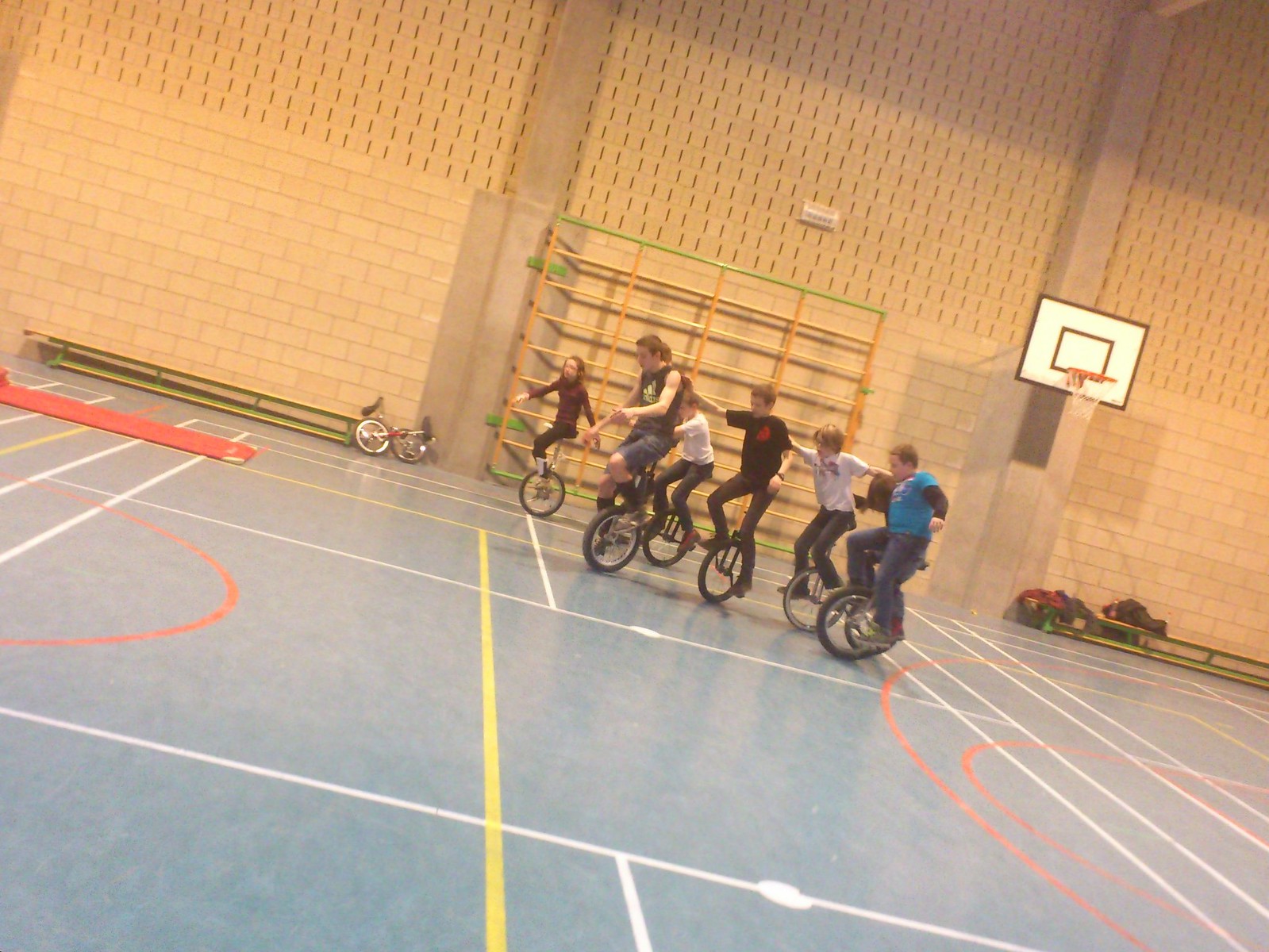The photograph captures a lively scene inside a gymnasium where a group of at least seven children are riding unicycles. The riders, mostly dressed in various colored t-shirts and jeans, are clustered together with many extending an arm to rest on a neighbor's shoulder or upper arm for balance and support. One rider, positioned in the background toward the left, notably rides alone without holding on to anyone. The gym floor is dark gray with basketball court markings and a visible hoop, unused unicycles scattered in the background. The shot, taken from a low right to upper left angle, gives the impression that the children are riding uphill. The gym features a brick wall with columns and is lit with yellowish lighting, adding a warm glow to the scene.